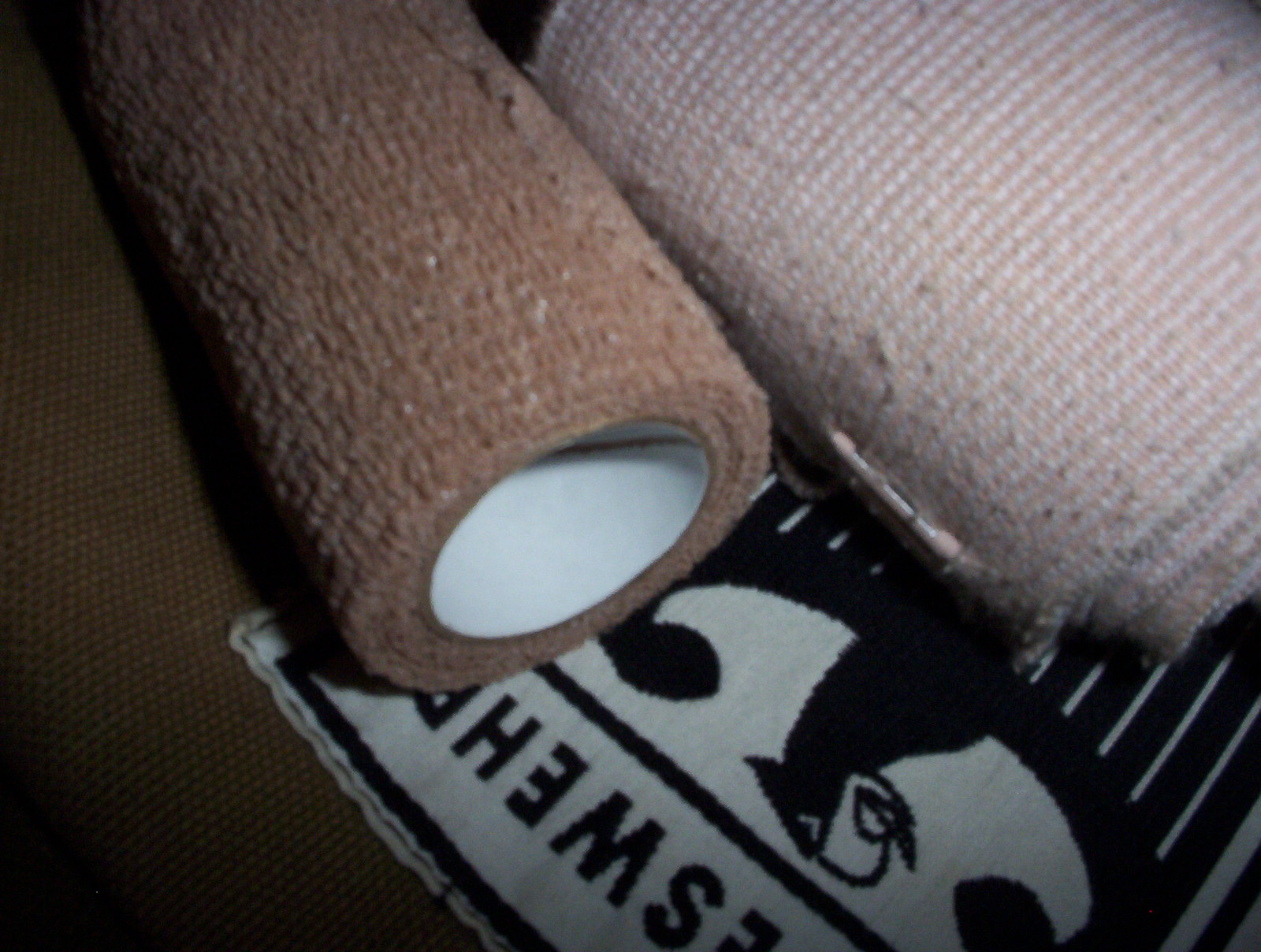The photograph captures a pair of medical bandages laid out side by side on a brown corduroy surface. The bandage on the far right is an ace bandage, used and re-rolled, exhibiting the typical light beige color and fabric texture associated with athletic wraps. On the left lies a dark brown self-adhesive compression bandage, about four inches wide, with a crêpe-like, tearable texture that allows it to stick to itself seamlessly. The corduroy fabric on which they rest features a partially visible black and white label with the letters "E-S-W-E-H-R" and a stylized eagle logo facing left, its feathers depicted by white slopes. This detailed and close-up image showcases not only the practical medical supplies but also hints at the possible setting, likely a personal item like a bag or a garment, providing both a functional and textured background.